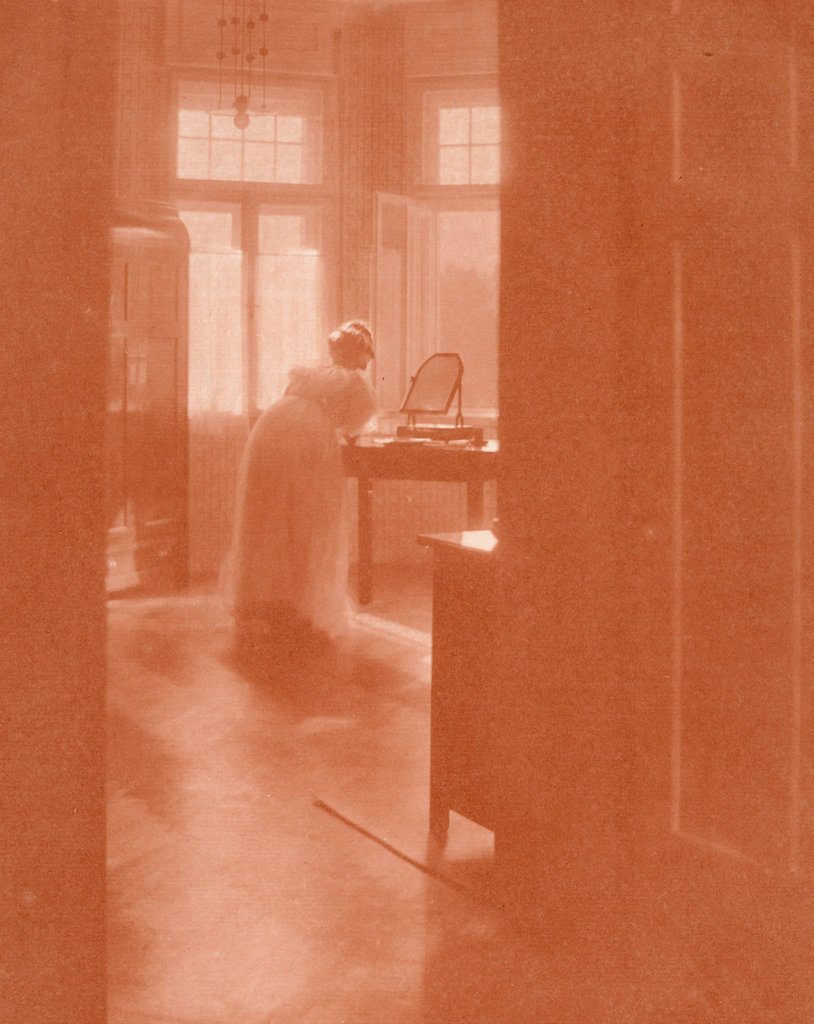In the image, which possesses a vintage, sepia-toned aesthetic reminiscent of early photography, a woman is captured in an elegantly lifelike pose that blurs the lines between photo and painting. She is positioned with her back to the viewer, facing a small mirror on a vanity table, as reflected in her profile. The scene unfolds within a room characterized by an open window, allowing natural light to cascade in, giving a warm, ethereal glow to the setting. The woman is adorned in a long, lacy, and flowy dress, indicative of a bygone era, adding to the nostalgic aura. Surrounding her, various objects such as a closet, a small lamp, and a door add depth to the room, all bathed in the predominant shades of brown, white, black, and gray. The wooden floor further anchors the image in its vintage appeal, making the scene both timeless and remarkably detailed in its simplicity and elegance.